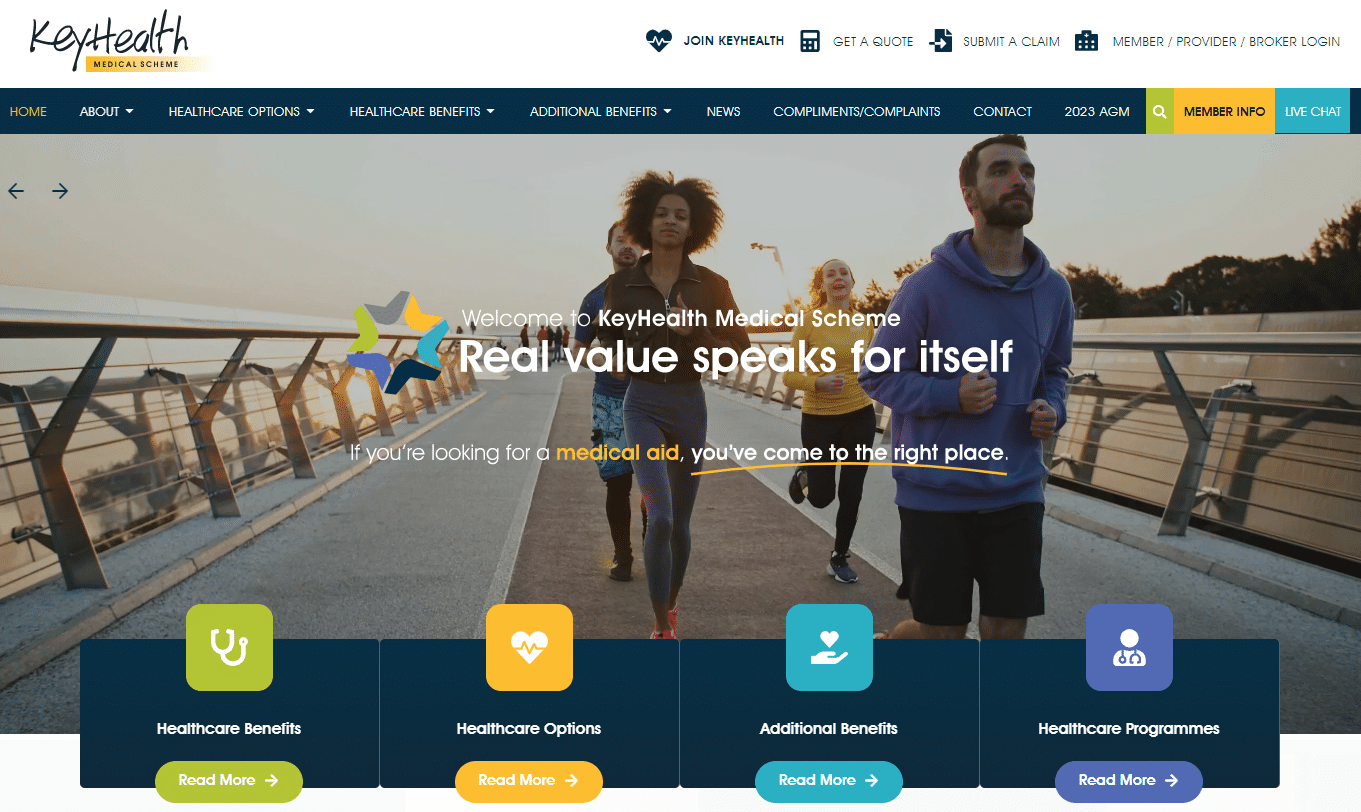The Key Health website provides comprehensive information about their medical scheme offerings. The homepage ("Home" tab highlighted in orange) features the Key Health logo alongside an image of a heart with a pulse, symbolizing their focus on joint health.

To the right of the logo, users can easily access key features including:
- A "Get a Quote" calculator.
- The option to "Submit a Claim," depicted by a document icon with an arrow.
- Login portals for "Members/Providers" and "Providers/Brokers," highlighted in orange.

Directly beneath this section, a blue navigation bar spans the width of the page, containing the following menu options:
- Home (highlighted in orange to indicate the current page)
- About (with a dropdown menu)
- Health Care Options
- Health Care Benefits
- Additional Benefits
- News
- Compliments/Complaints
- Contact
- 2023 AGM (Annual General Meeting)

On the right end of this bar, there’s a green background with a magnifying glass icon labeled "Search" and an orange tab labeled "Member Info." Additionally, a blue tab for "Live Chat" is available for immediate assistance.

Below the navigation bar, there is a vibrant image of four runners on a road bordered by guard railings. The runners include a woman with large curly hair and leggings, a man in a hoodie leading, and a white woman with long sleeves behind them.

The welcoming message, "Welcome to Key Health Medical Scheme, real value speaks for itself," is prominently displayed, followed by quick access links to:
- Health Care Benefits ("Read More" in green)
- Health Care Options ("Read More" in orange)
- Additional Benefits ("Read More" in light blue)
- Health Care Programs ("Read More" in dark blue)

Each link invites the user to explore more detailed information about the specific offerings available under the Key Health Medical Scheme.